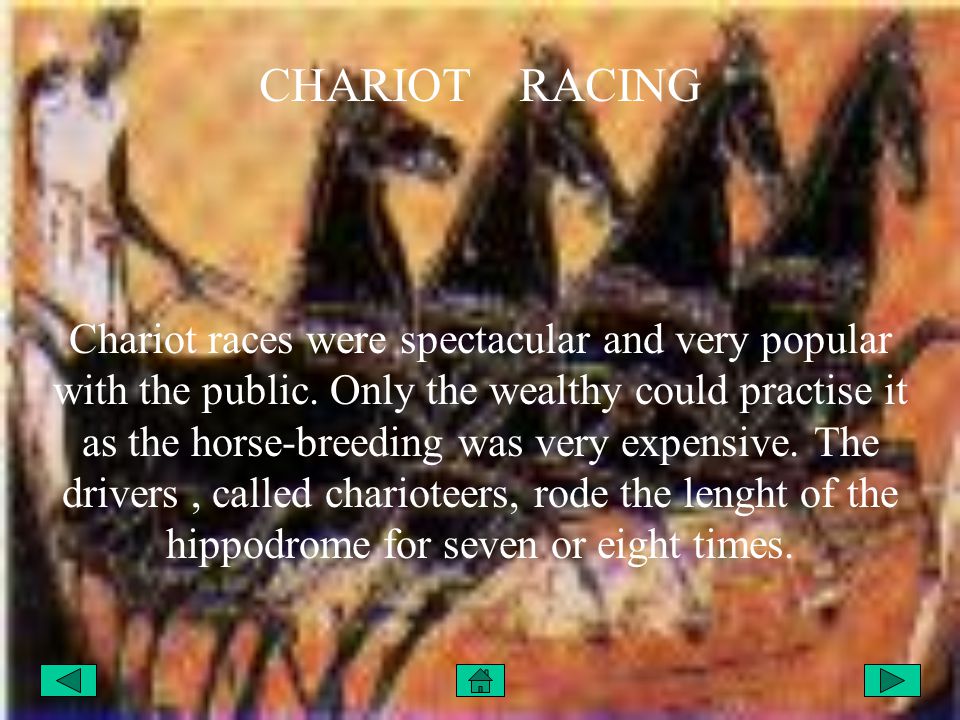The image depicts a presentation slide, primarily in warm orange tones with a blurred background, illustrating chariot racing. Dominating the imagery is an Egyptian-style painting or drawing featuring four black horses pulling a chariot driven by a figure in white robes. This figure holds the reins firmly as the chariot races forward. Prominently displayed in white text, the title reads "Chariot Racing" with an informative blurb that follows: "Chariot races were spectacular and very popular with the public. Only the wealthy could practice it as horse breeding was very expensive. The drivers, called charioteers, rode the length of the hippodrome for seven or eight times." The slide interface includes green navigation buttons: a left-facing arrow, a home button, and a play button, suggesting the content is part of a digital presentation or webinar.